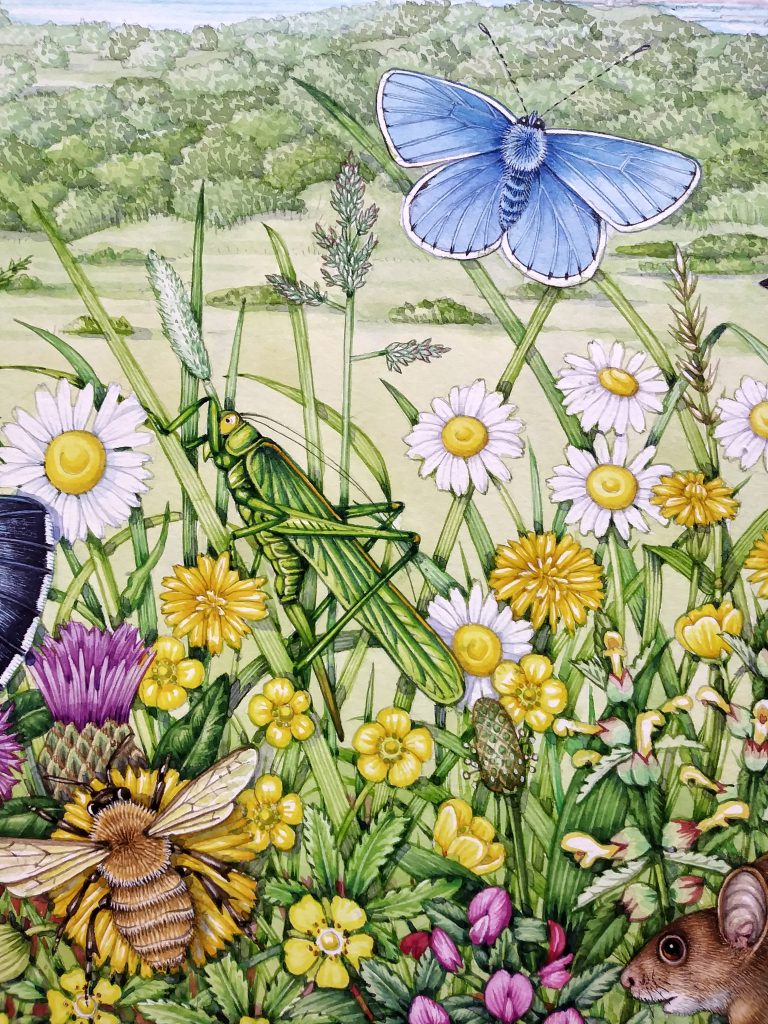This artwork is a vivid and detailed painting of a blooming garden set against a lush, hilly landscape. At the top of the image, a small sliver of blue hints at either a distant sky or water, framed by varying shades of green that depict tree-covered hills. In the foreground, a vibrant array of flowers takes center stage, including bright yellow sunflowers, white daisies with sunny centers, and a few pinkish-purple blooms. Amongst the flowers, a large blue butterfly with white-edged wings and a furry blue center prominently flutters above.

To the far left, a big yellow and brown bumblebee perches on a yellow flower. On the right, a small animal, resembling a mouse with a big ear and a shiny beady eye, peeks out from the corner of the scene. Not far from it are some pinkish-purple flowers. Toward the middle but slightly to the left, a green grasshopper is seen clinging to a stalk of grass. This close-up view of this patch of grass also captures various other insects, making the entire garden scene teeming with life and color, while the background gradually transitions into grasses and trees on distant hills.